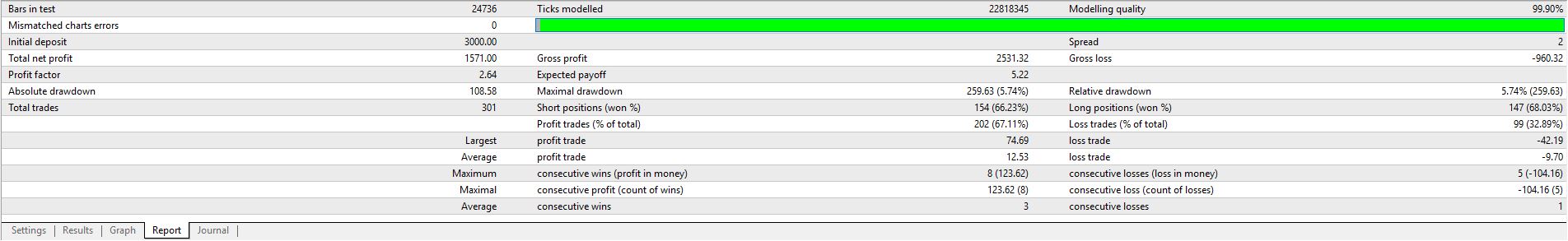The image depicts a detailed financial report, typical of what one might find in accounting software like QuickBooks. The report is presented in a table format with alternating bands of light gray and white for ease of reading. 

- In the top-left corner, the heading reads "Bars and Tests," followed by the numeric identifier "24736."
- Below this, the entry "Mismatched Charts Errors" is recorded as "0."
- "Initial Deposit" is listed as "$3,000."
- "Total Net Profit" is stated to be "$1,571."
- The "Profit Factor" is calculated at "2.64."
- The "Absolute Drawdown" is noted as "108.58."
- "Total Trades" conducted are "301."

Further detailed financial metrics include:
- "Largest Average, Maximum, Maximal, and Average" statistics are shown.
- "Ticks Modeled" is represented by a green rectangle stretching completely from left to right.
- "Gross Profit" is listed as "$2,531.32."
- "Expected Payoff" is marked at "5.22."
- "Maximum Drawdown" stands at "259.63."

Position-specific data:
- "Short Positions" are shown as "1, 154."
- "Profit Trades" percentage of total is "202."
- "Profit Trade" entries are "$74.69" and "12.53."
- "Consecutive Wins (Profit and Money)" lists "8."
- "Consecutive Profit (Count of Wins)" is "123.62."
- "Consecutive Wins" total "3."

Quality and loss-related data:
- "Modeling Quality" shows "99.90%."
- "Spread" is "2."
- "Gross Loss" is recorded as "$960.32."
- "Relative Drawdown" is "5.74%."
- "Long Positions" reported are "1, 147."
- "Lost Trades" total "99."
- "Lost Trade" values are "-42.19" and "-9.70."
- "Consecutive Losses (Loss and Money)" count "5."
- "Consecutive Loss (Loss of Losses)" details a total loss of "-104.16."
- "Consecutive Losses" are at "1."

The structured layout and comprehensive details provide a thorough financial snapshot, highlighting both profits and losses across various metrics.